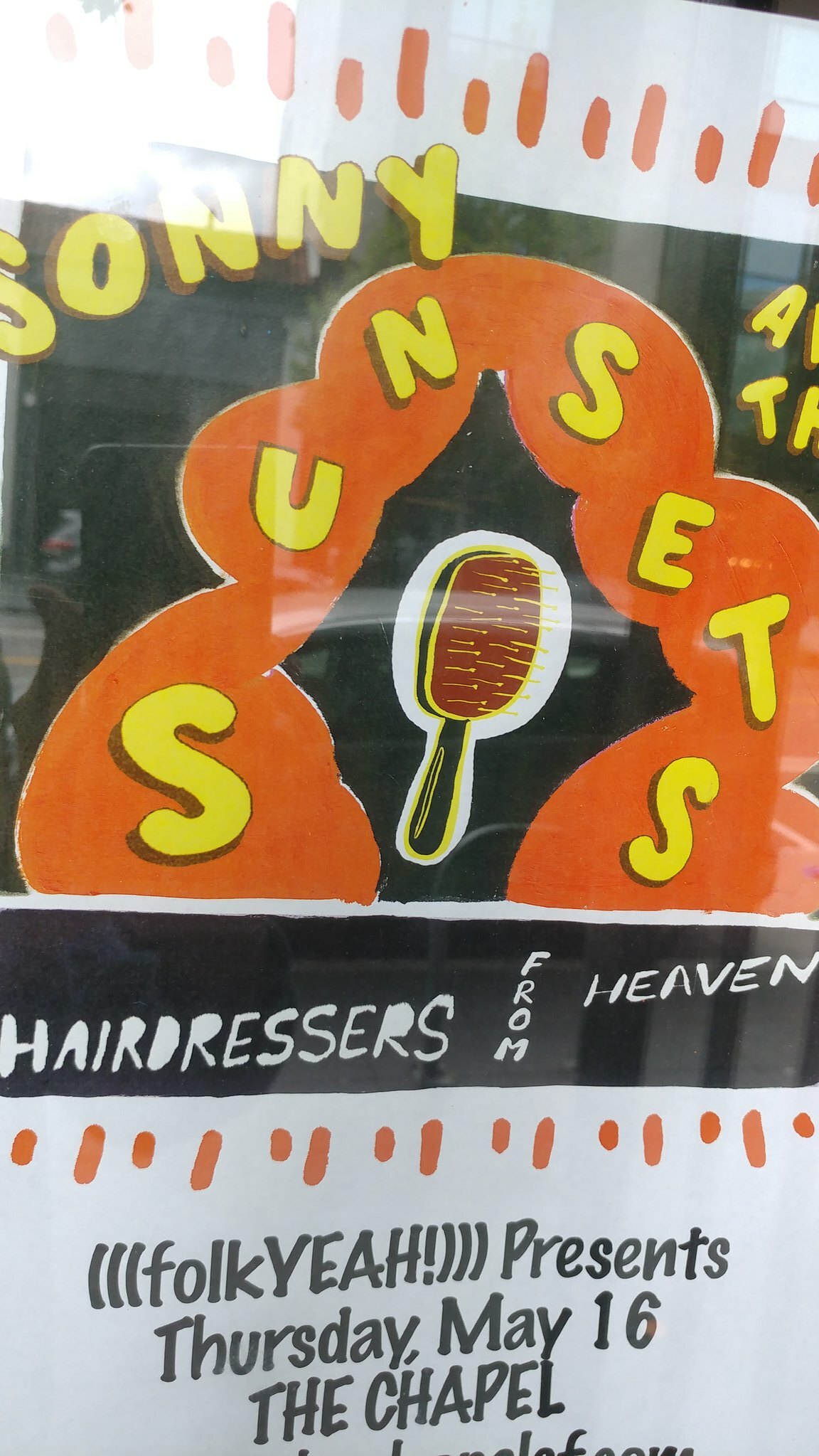The image depicts a hand-drawn poster displayed on the other side of a window, creating a reflection that shows parts of the street and nearby buildings. The poster has a white bar at the top with small vertical orange lines. Below this, against a black backdrop, the word "SUNNY" is prominently displayed in yellow puffy font, spelled out "S-O-N-N-Y" like someone's name. Just beneath, in a circular arrangement surrounding an image of a black hairbrush with yellow bristles, the word "SUNSETS" is written in yellow letters. A black bar below this reads "HAIRDRESSERS FROM HEAVEN" in white ink. Further down, another section with a white background and black letters announces "Folk, Yeah! presents Thursday, May 16th, The Chapel." The artistic design and color scheme emphasize the eye-catching and creative nature of the poster.